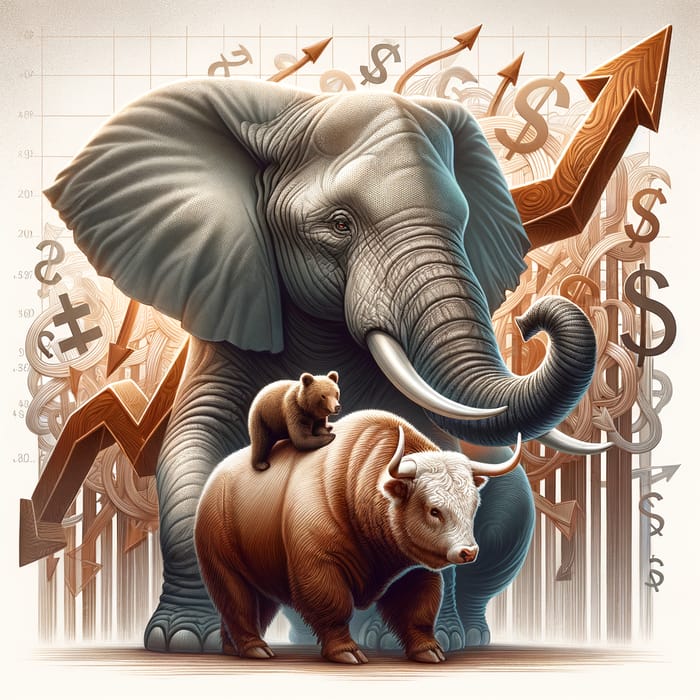The image depicts a large gray elephant with prominent white tusks at the center. In front of the elephant stands a brown bull with a white face and sharp horns. Clinging onto the bull's back is a tiny brown and black bear cub, seemingly holding on for dear life. The background features an intricate pattern of brown and gray arrows and dollar signs, resembling a numerical graph paper. The color scheme consists of neutral shades, predominantly blue, brown, black, white, and beige. This graphic illustration symbolizes political and financial influences on the stock market, with the animals possibly representing different market forces amidst a backdrop of financial data and trends.